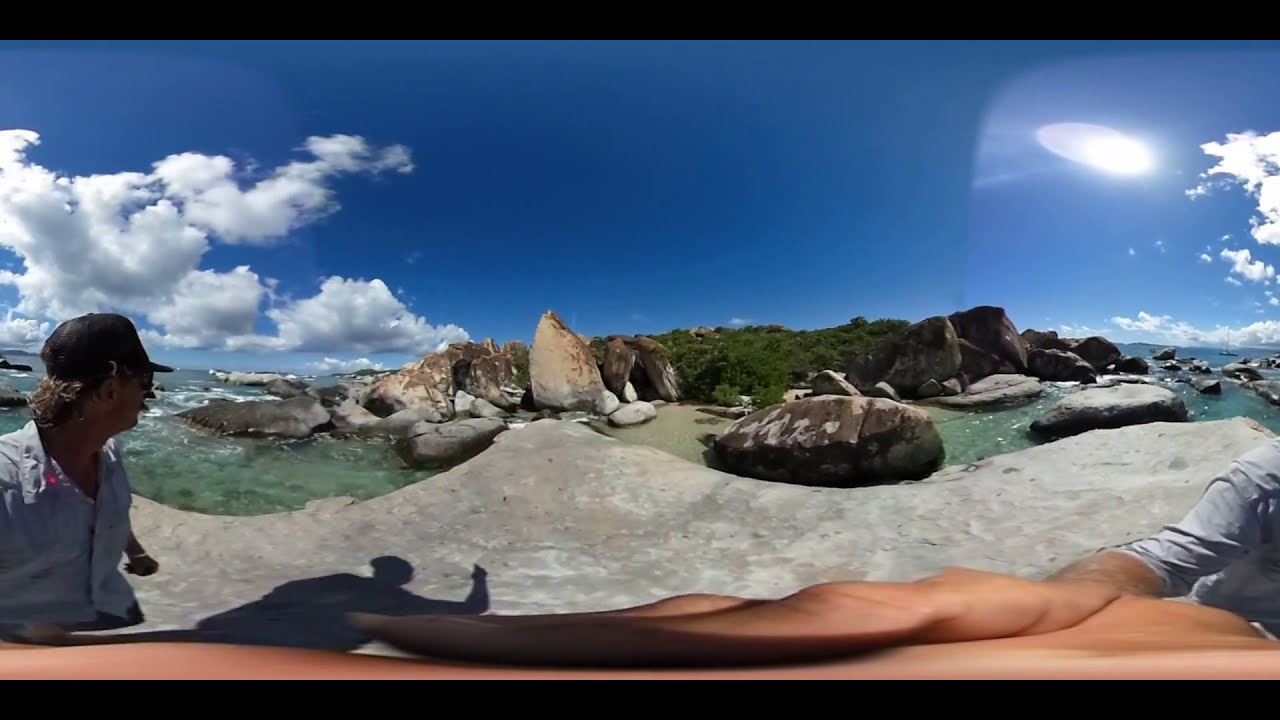The image showcases a panoramic view of a waterfront area with a man in a black baseball cap and long, neck-length hair standing near the water. He is wearing a slightly popped-collar, blue shirt and is positioned towards the left half of the image, looking to the right. His face is obscured by shadows. The man’s left hand is clenched into a fist and adorned with a bracelet. 

Another hand, noticeably wide and occupying the left-to-bottom corner of the image, belongs to a person in a short-sleeved, gray shirt. This hand appears to be holding the camera, contributing to the panoramic effect. 

The landscape features a mix of large stones and boulders scattered across the water, with white suds floating among the rocks indicating wave activity. Some rocks are as large as the people in the image, and one boulder particularly resembles the top half of a boat. There is a sandy patch in the center of the view, leading to a small concrete pathway or ramp that descends to the water. Surrounding the water are dense patches of green shrubbery and trees, situated on a small hill.

In the background, the sky transitions from clear blue in the center to areas with fluffy white clouds accented with gray tones on the left. On the right side of the image, the sun is visible among more clouds. A sailboat can also be seen in the distance to the right. The water itself reflects a serene mix of green and blue hues.